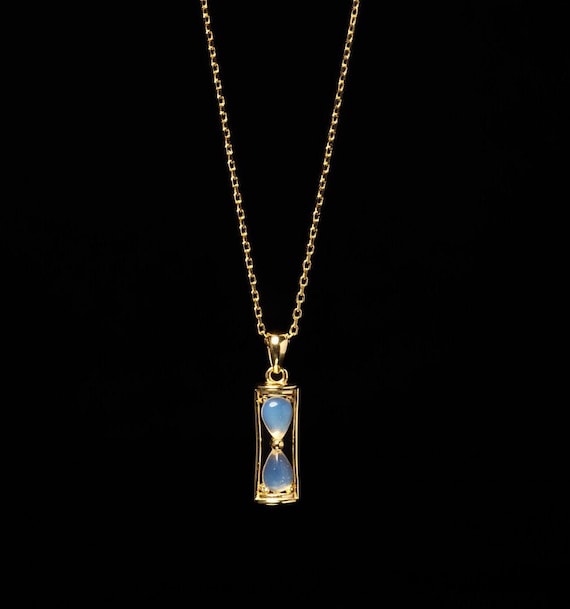The image features a luxurious, dainty necklace crafted from what appears to be 14-karat gold, gleaming brightly against a stark black background. The centerpiece of the necklace is a unique hourglass-shaped pendant, composed of two smooth, light blue gemstones. Each gemstone is meticulously set within a golden, rectangular frame that tapers elegantly at the center, accentuating the hourglass design. The pendant is suspended from the chain via a refined gold ring, adding a touch of simplicity to the intricate design. The overall composition highlights the exquisite craftsmanship and the striking contrast between the glowing gold and the serene blue gemstones.